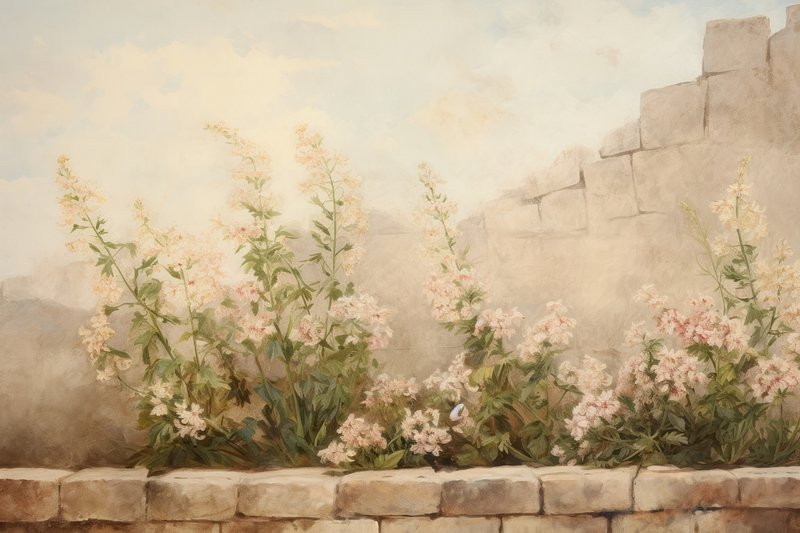This detailed painting vividly captures a scene featuring a flower pot constructed along the side of a building. The base of the image showcases a stone wall made of pinkish, grayish beige bricks. Above this wall, verdant green foliage and light pink or peach flowers flourish, extending across the entire width of the painting, from the left side to the right edge. These flowers have green stems and are depicted in various positions—some ascending, some reaching to the left, while others grow straight up or lie near the ground. In the background, another stone wall is visible, appearing taller and extending from the middle of the image up towards the top right corner. This background wall has a more faded, gray appearance, blending into an atmospheric backdrop filled with hints of fog or smoke. To the left of the flowers, faint outlines of hills can be discerned, merging into a hazy mix of gray and brown shapes. Overhead, the sky is a mix of blue with white and gray clouds, adding a serene touch to this highly detailed and textured artwork. Notably, the image contains no text.